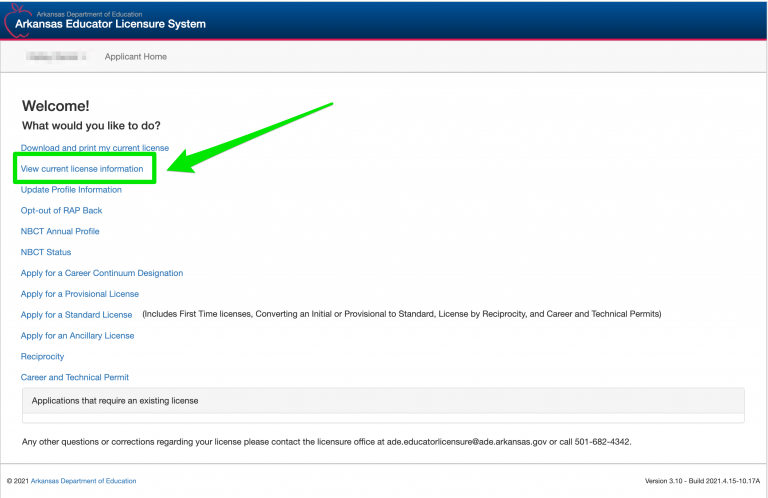In this image, we see a landing page for an education website, specifically for the Arkansas Department of Education's Arkansas Educator Licensure System. The top section features a blue header that prominently displays the title alongside a logo that outlines an apple. Below this, the screen transitions to a white background with the heading "Applicant Home."

Underneath this heading, there is a welcoming message on the left side of the screen in black text that asks, "Welcome. What would you like to do?" Following this, a list of options is presented in light blue text. These options include "Download and print my current license," and "View current license information," with the latter being highlighted by a green circle and an accompanying green arrow pointing to it. Below these, additional options are listed: "Update profile information," "Opt out," "RIP back," "NBCT Annual Profile," "NBCT Status," "Apply for a career continuation designation," "Apply for a provisional license," "Apply for a standard license," "Apply for an ancillary license," and "Reciprocity Career and Technical Permit." The overall layout is organized to help users easily navigate through various licensure-related tasks.